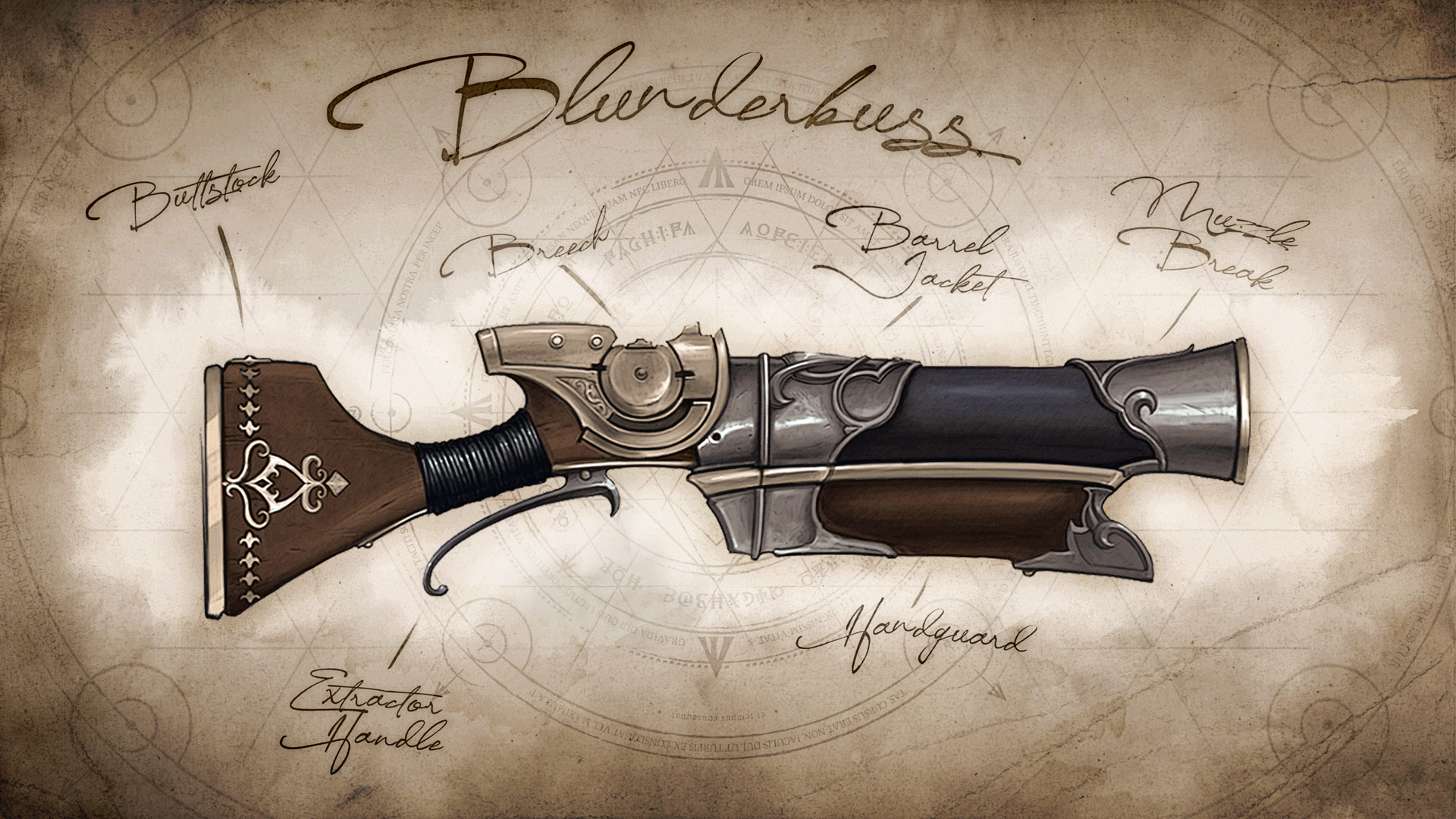The image features a detailed hand-drawn piece of art centered around an exaggerated, slightly cartoonish rifle reminiscent of those found in fantasy or steampunk fiction. The rifle itself, labeled "Blunderbuss" in hand-drawn cursive text above it, showcases a mix of colors: silver at the barrel, transitioning to black, and then silver again, with the chamber around the bullets depicted in gold. The handle and buttstock are crafted to appear wooden with a brown base, adding to its whimsical aesthetic.

Above different parts of the rifle, there are annotations in the same cursive text, such as "buttstock" toward the rear and other terms like "barrel jacket," "exhausted," "exhaust handle," and "handle card," pointing to various components. The trigger of the rifle is silver, adding a consistent metallic detail.

The background enhances the antiquated feel of the piece, featuring sepia tones reminiscent of old parchment. It is adorned with Latin-like lettering and arcane drawings, suggesting an ancient or mystical theme, as though the artwork was rendered on a weathered map or piece of old paper. This setting reinforces the fantastical and timeless nature of the rifle illustration.